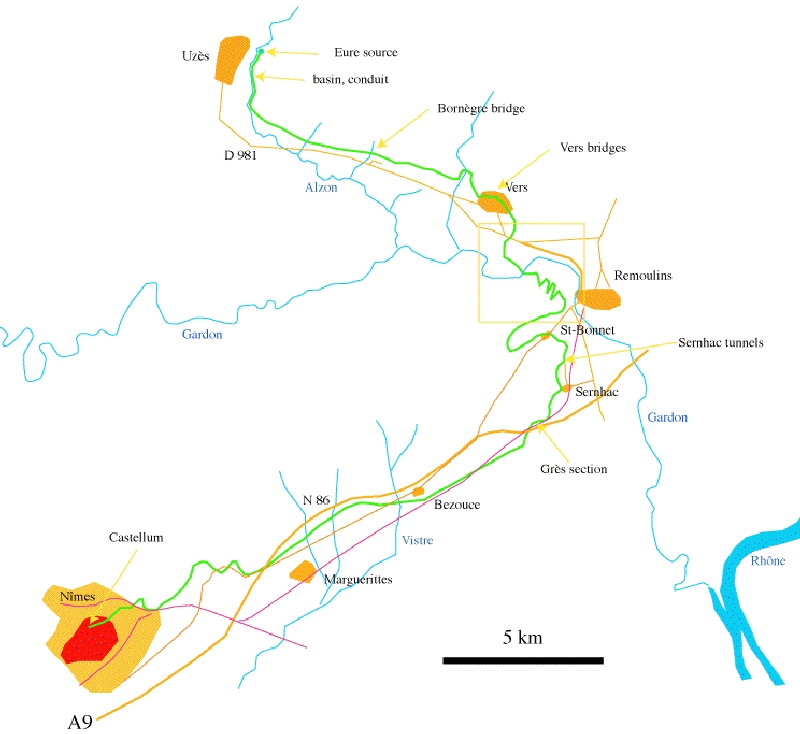This digital map features multiple color-coded lines representing waterways or rivers, all set against a white background. Prominently, light blue lines labeled with names such as 'Gardon' and 'Alzon' indicate major waterways. Yellow lines, annotated with terms like 'source,' 'conduit,' 'bridge,' 'verse,' and 'remulans,' seem to highlight various infrastructure elements and locations like 'saint bonnet' and 'serhac.' A dark orange line, a lighter orange line, and a green line squiggle across the map, converging into an orange and red section towards the bottom left. These colored lines have arrows pointing to them, with some corresponding to previously mentioned names. Additionally, a dark yellow line and a squared-off area, both with arrows and labels, are present. Importantly, a yellow shape with a red core is marked 'castellum,' with references to 'nimes' and 'a9.' At the bottom right of the map, a legend indicates that a black line denotes a 5-kilometer distance for scaling.